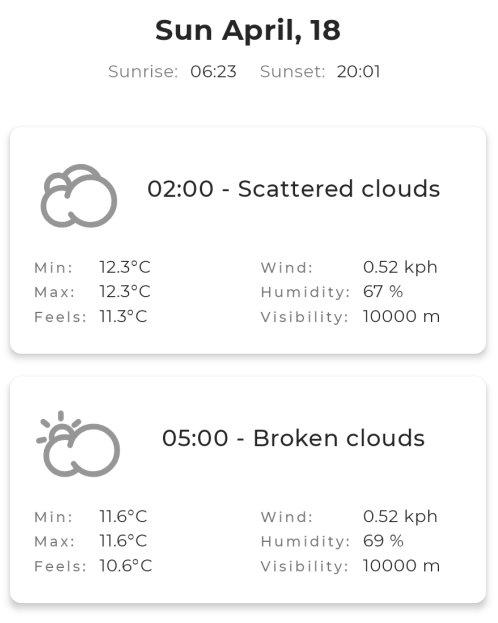The image consists of two horizontally-aligned white boxes with pale gray borderlines, stacked one on top of the other, set against a white background. Each box provides weather reports for a Sunday, specifically April 18th, as noted at the top of the image in bold black text "Sun, April 18." Just below this, in gray text, are the times for "Sunrise: 6:23" and "Sunset: 20:01."

In the first box, on the left, there is a gray-outlined cloud icon, indicating cloud coverage. To the right of this icon, the text reads "2 o'clock - Scattered Clouds." Below this, the weather details are listed in light gray text: "Min: 12.3°C, Max: 12.3°C, Feels like: 11.3°C, Wind: 0.52 kph, Humidity: 67%, Visibility: 10,000m."

In the second box, there is another cloud icon, but this time with the sun partially visible behind it, symbolizing partly cloudy conditions. To the right of this icon, in black text, it reads "5 o'clock - Broken Clouds." Below this, similar weather details are provided: "Min: 12.3°C, Max: 12.3°C, Feels like: 11.3°C, Wind: 0.52 kph, Humidity: 67%, Visibility: 10,000m."